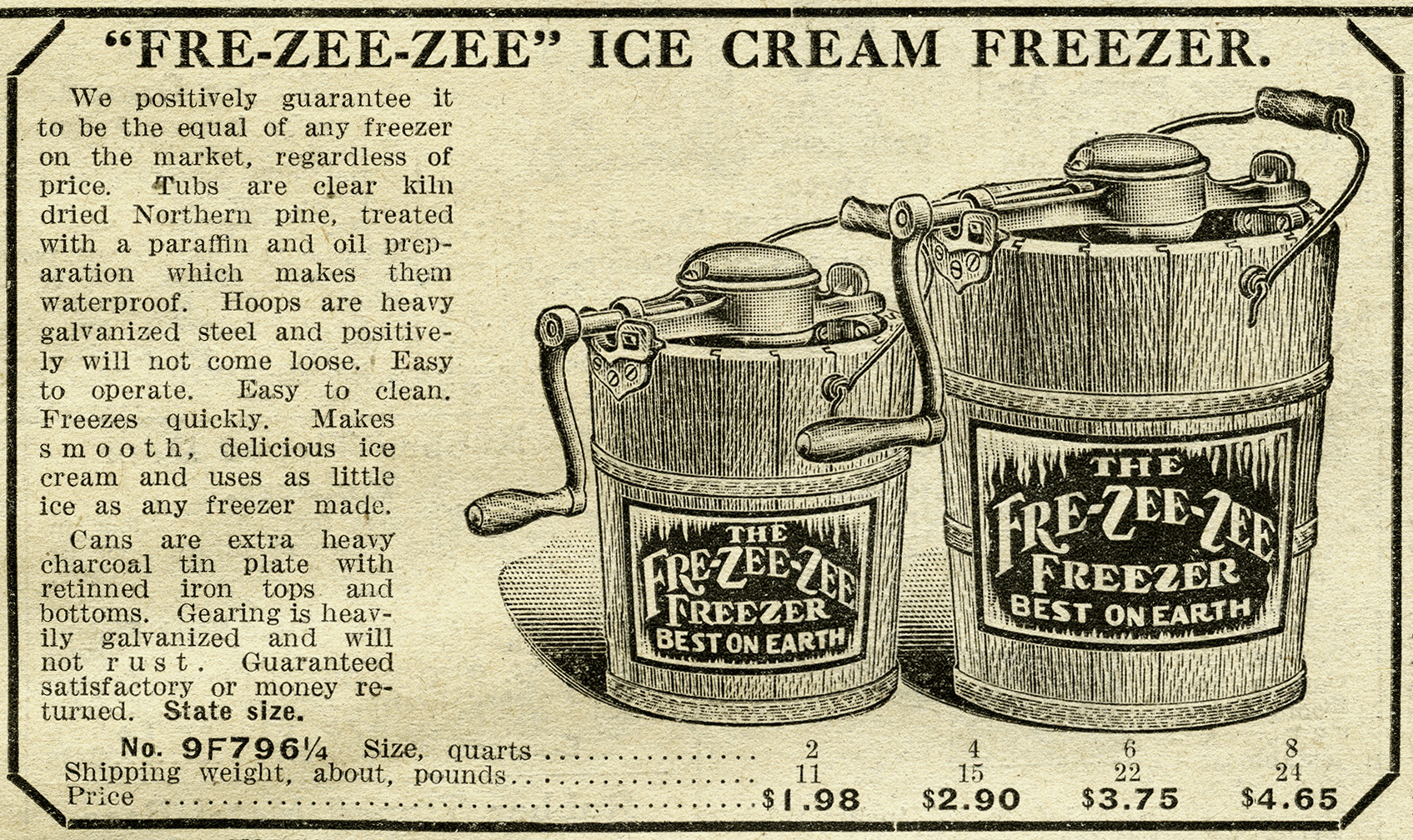This vintage advertisement showcases the "Free ZZ Ice Cream Freezer," a manual ice cream maker. The ad features two prominently displayed ice cream freezers, resembling wooden buckets outfitted with galvanized steel bands and a metal contraption on top, complete with a hand-crank for churning. Made from kiln-dried northern pine treated with a waterproof paraffin and oil preparation, these freezers are touted for their durability and efficiency.

The ad details multiple sizes available—2, 4, 6, and 8 quarts—with corresponding shipping weights of 11, 15, 22, and 24 pounds, and prices set at $1.98, $2.90, $3.75, and $4.65 respectively. The label on each freezer boasted it as "The Free ZZ Freezer—Best on Earth," and the product is guaranteed to match the quality of any freezer on the market. The heavily galvanized gearing is advertised as rust-resistant, promising smooth, delicious ice cream with minimal ice usage. The ad emphasizes the product's ease of operation and cleaning, with a hefty endorsement: "Guaranteed satisfactory or money returned."